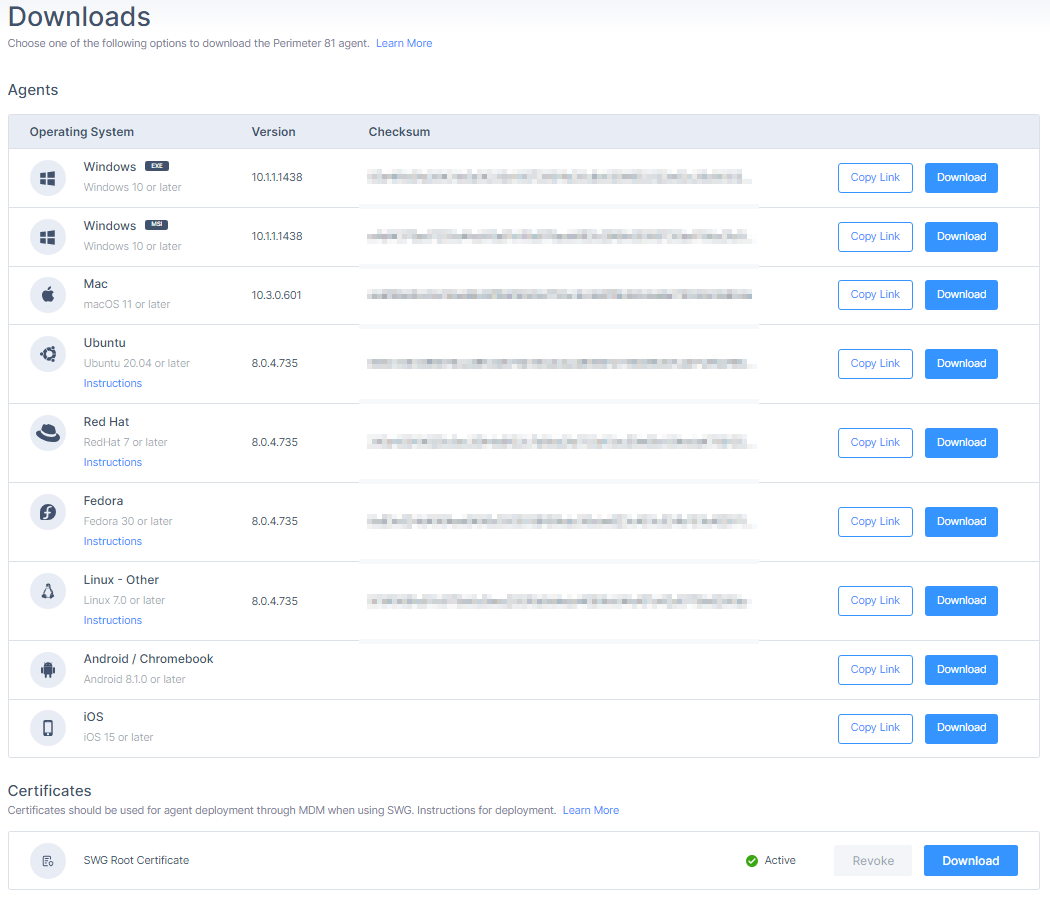The image is a screenshot of a Downloads page for the Perimeter 81 agent, featuring various options for downloading the software. At the top of the screenshot, the title "Downloads" is prominently displayed. Below this title, there's a prompt inviting the user to "choose one of the following options to download the Perimeter 81 agent," accompanied by a "Learn More" link in blue text. 

The text appears in a small font size. Further down, the section is labeled "Agents," followed by a blue horizontal stripe with the label "Operating System" on the left side. To the immediate right of "Operating System," there are column headers labeled "Version" and "Checksum."

Beneath the "Operating System" header, there is a detailed list of supported operating systems and their corresponding versions:

1. **Windows**: Windows 10 or later
2. **Windows**: Windows 10 or later
3. **Mac**: macOS 11 or later
4. **Ubuntu**: Ubuntu 20.04 or later, followed by a blue "Instructions" link
5. **Red Hat**: Red Hat 7 or later, followed by a blue "Instructions" link
6. **Fedora**: Fedora 30 or later, followed by a blue "Instructions" link

Each operating system entry includes a small circle with a symbol inside it, possibly indicating an icon or download button.